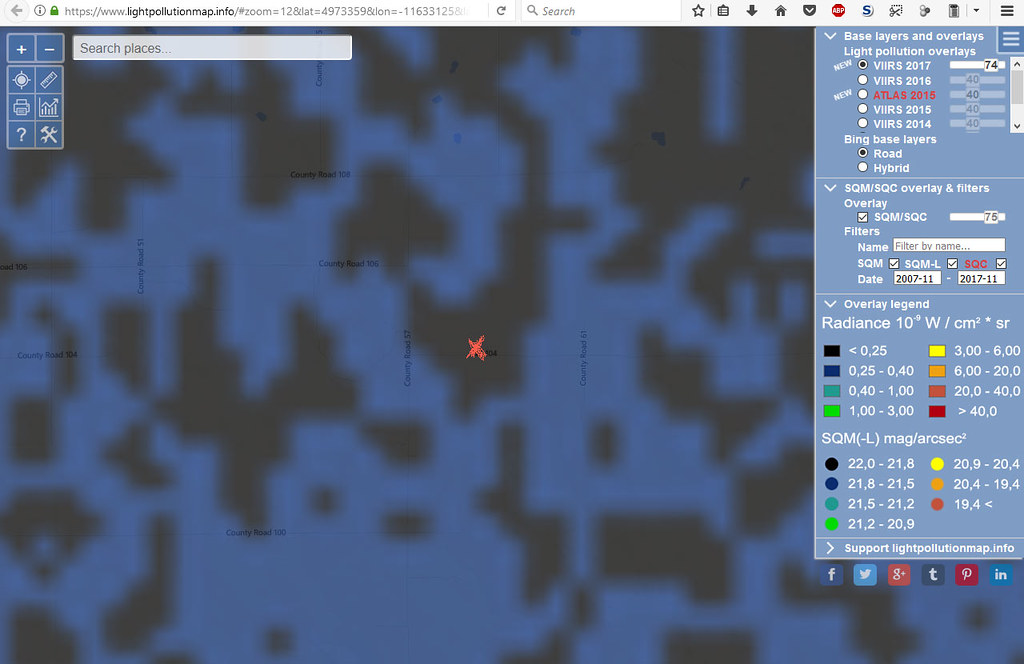**Caption:**

The image showcases a computer screen displaying a digital map interface. At the center of the screen lies a small red "X" marker, surrounded by black grid-like areas and blue sections resembling puzzle pieces. In the upper left corner, a series of functional icons can be seen, including a plus sign, likely for zooming in, a minus sign for zooming out, a compass, a ruler, a printer image, a graph icon, a question mark, and a tool icon. The map, characterized by its blue background and black grid squares, spans the majority of the screen.

On the right side of the interface, multiple adjustment options are available, including layer management, filter and overlay customization, and color adjustments. These features suggest that the image is of a map editing and customization tool. At the bottom of these editing options, several social media icons are visible, including Facebook, Twitter, Google Plus, Pinterest, and LinkedIn, indicating sharing capabilities.